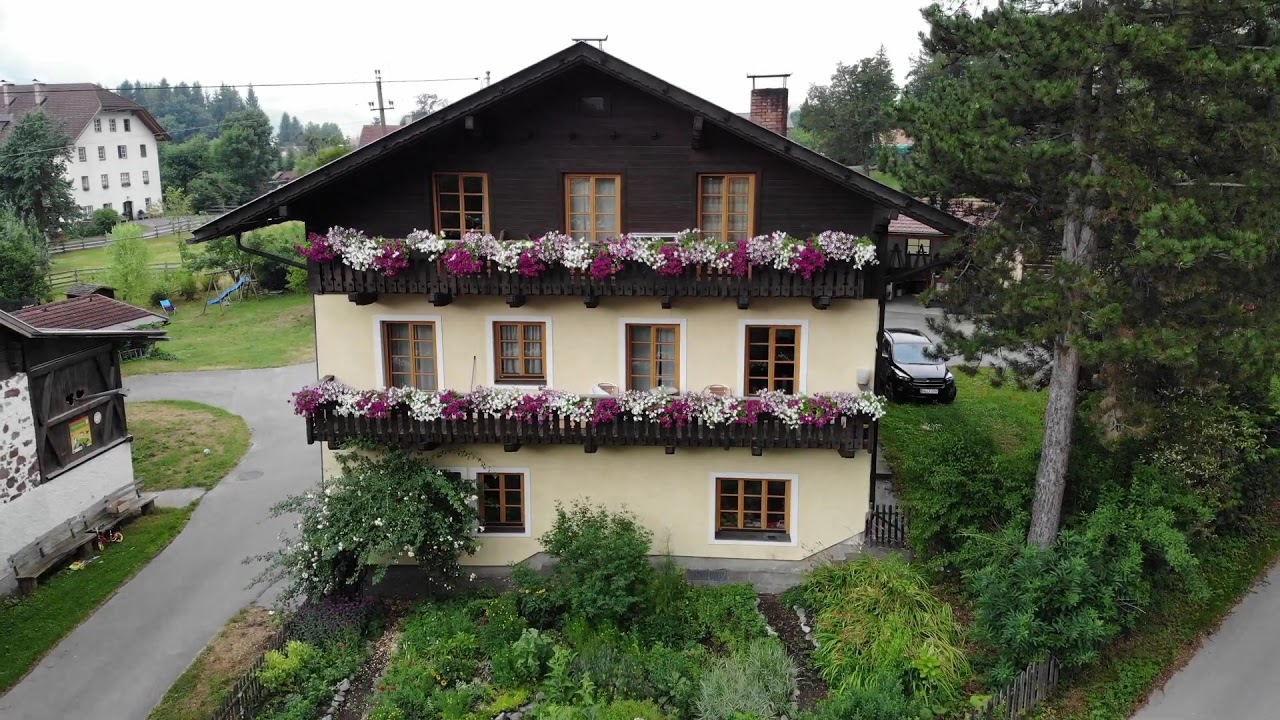In a somewhat overcast, slightly cloudy sky, a serene residential area unfolds with a vivid picture of a charming three-story house prominently featured. The house boasts a distinctive color palette with the bottom two floors in a cream or tan hue, contrasted by a dark brown third floor topped with a matching brown roof. The side or front of the house, facing the viewer, is adorned with two picturesque balconies on the first and second floors, each blooming with a mix of purple, white, and occasionally red flowers. Light wood trims accentuate numerous windows: two on the ground floor, four on the second floor, and three on the third floor.

In front of the house, bright green bushes and trees cluster, their foliage extending to the right side of the building. To the left, a smaller, mixed white and brown building stands nearby, separated by an asphalt path. Nearby, a dark sedan is parked.

Further into the background, a three or four-story structure with a uniquely slanted brown roof is visible among more trees and light green grass. Additional power lines, smaller thin trees, and a network of paths—including a secondary road to the bottom right—stitch this idyllic setting together, enhanced by the charm of a potential farm-style house peeking in the distance.